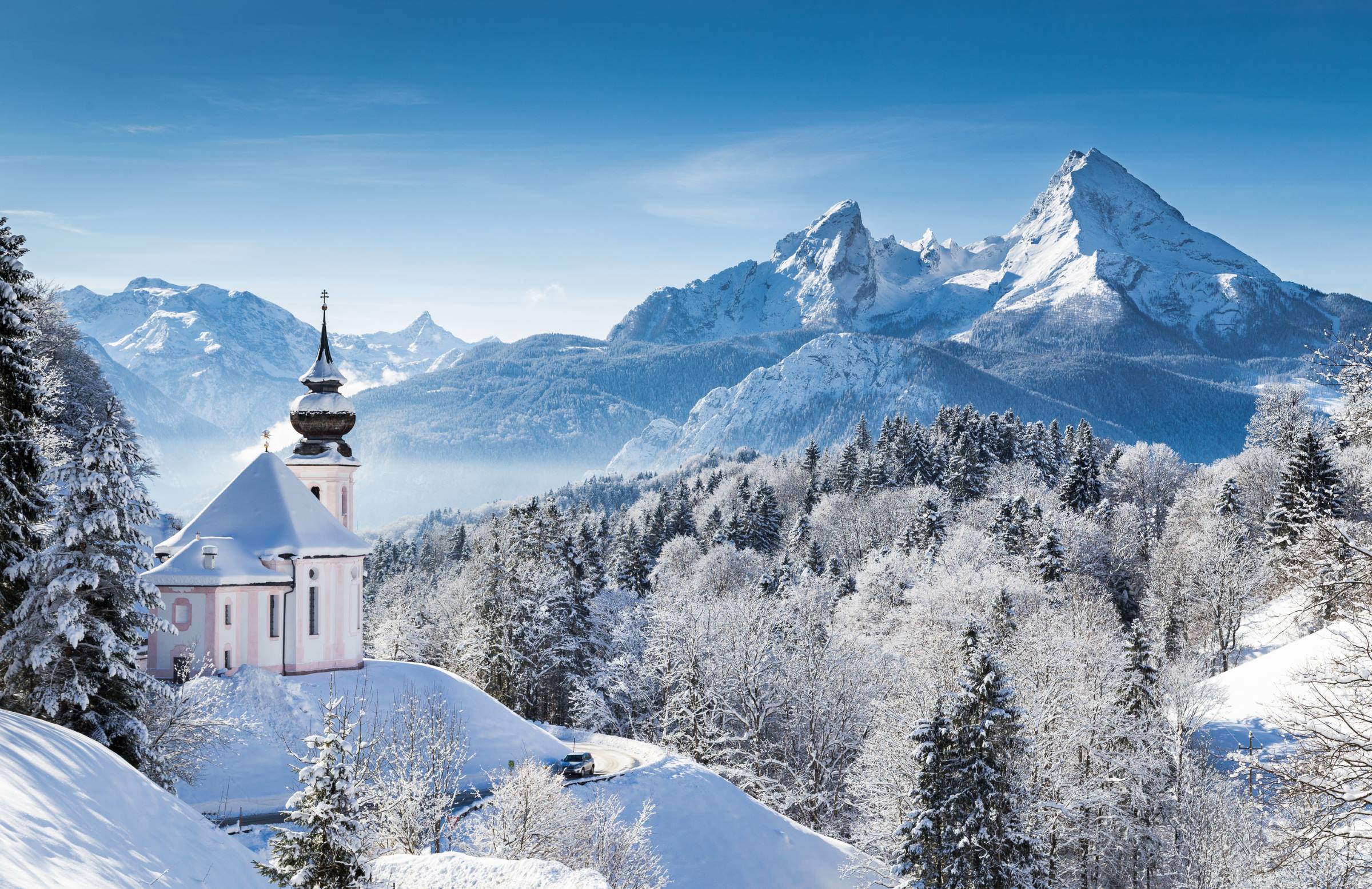A breathtaking photograph captures a serene winter landscape dominated by a snow-covered, white structure on a hillside, resembling both a church with steeples and an elegant house with a blue roof. This stunning building, reminiscent of a small castle with a cylindrical tower, stands majestically against a backdrop of jagged, snow-capped mountains under a bright blue sky dotted with wispy white clouds. A winding road curves around the hill, and a distant car is barely visible beneath the blanket of snow. Snow-laden green trees border the scene, adding to the picturesque setting, which could be in Vermont or the Swiss Alps. The entire landscape, from the pristine building to the vast grove of white-covered trees, exudes a peaceful, almost enchanting winter charm.